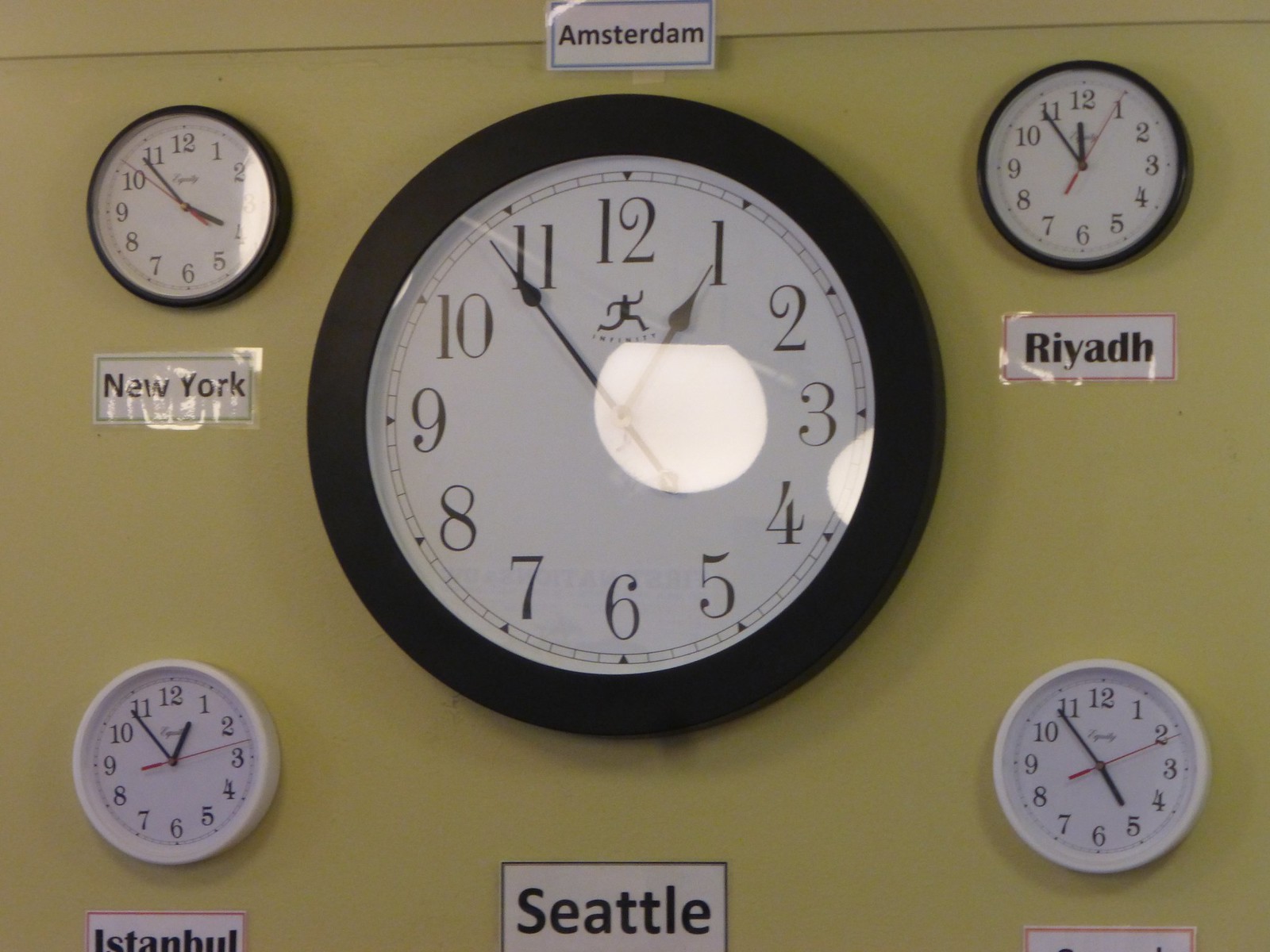The image depicts a collection of five clocks arranged on a yellowish-green or possibly discolored white wall. Each clock is tagged with a laminated piece of white paper, displaying the name of a different global city in black lettering. 

Centrally positioned on the wall is a large, circular clock with a thick black frame. It is marked "Seattle" beneath it, showing the time as 1:09. Situated to the top right of this central clock is a smaller clock, approximately a quarter of the size of the central clock, labeled "Riyadh" with the time displaying 11:55.

In the bottom right corner of the arrangement, another smaller clock, similarly sized to the Riyadh clock, is partly out of frame. Despite this, it shows the time as either 5:54 or possibly 1:54. 

To the bottom left of the central clock is another small clock labeled "Istanbul." This clock’s hands point to either 1:54 or 12:54, making it hard to discern precisely.

Above the central large clock is a label marked "New York," with a smaller clock hanging above it showing either 3:54 or 4:54. Over to the top of the scene, a label reading "Amsterdam" implies that the primary large clock might belong to Amsterdam, suggesting that the "Seattle" label could correspond to another clock situated beneath this main clock.

The arrangement on the wall creates a global tableau, each clock presenting the current time in major cities across different time zones.